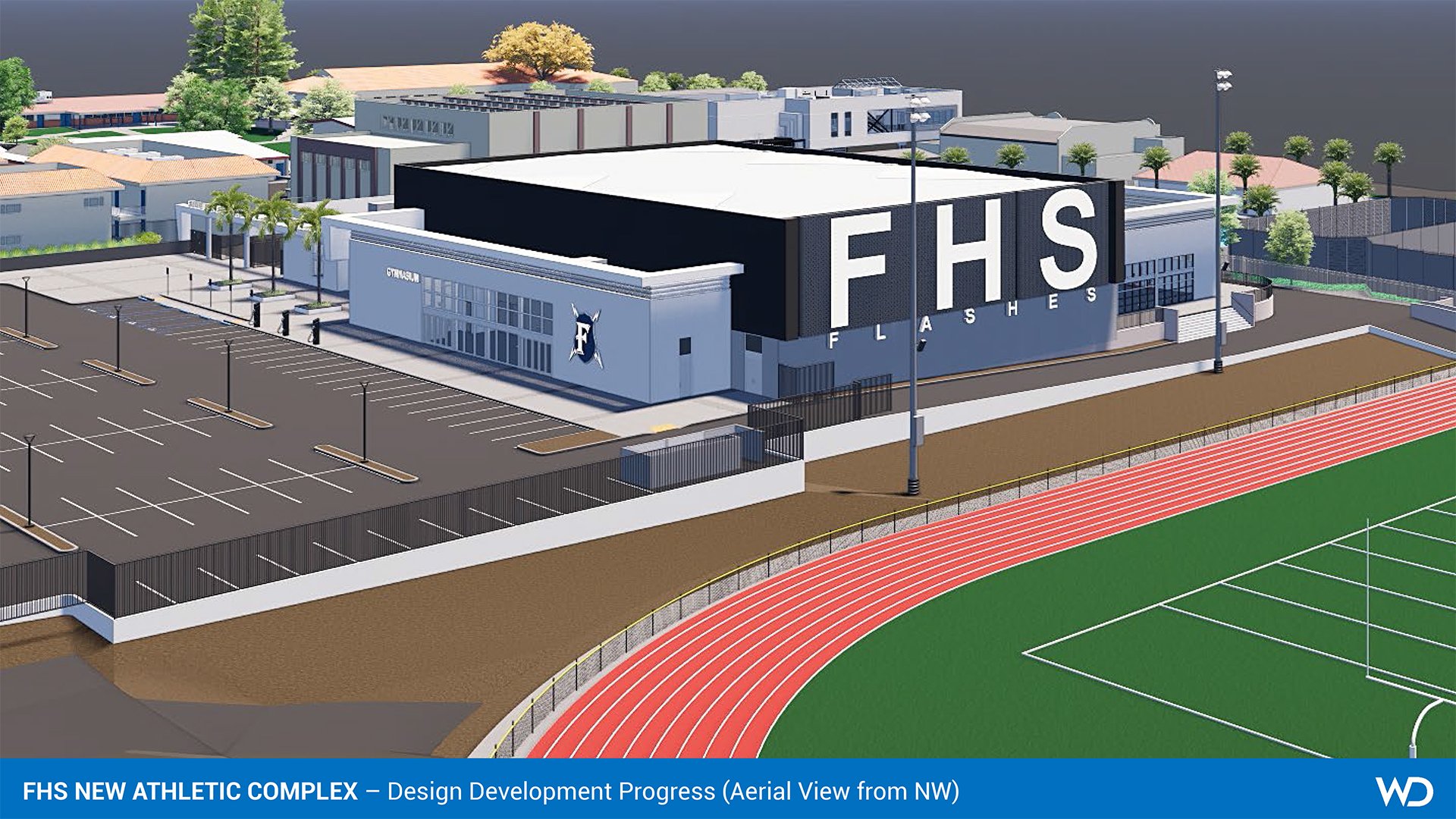This computer-generated image depicts the proposed design of a new athletic complex potentially for Flashes High School. Central to the image is an angular, white-walled building adorned with the large, white letters "FHS" across the front facade, and "Flashes" beneath. To the left of this building lies a large parking lot, likely intended for student use, featuring a brownish-gray surface. Surrounding the building, the background fades to a homogeneous gray, offering no clue whether it is day or night, while a mixture of trees, including palm trees, suggests a southern locale.

Occupying the lower right section of the image is an expansive athletic facility. A running track with nine lanes, marked in red, encircles a green football field complete with visible lines and goal posts. Adjacent to this track is a fenced-off gray dirt area, enhancing the functional layout of the complex. Notably, the bottom section of the image features a distinct blue bar containing white text that reads, "FHS New Athletic Complex," with a subtitle, "Design Development Progress," and a parenthetical note, "Aerial View from NW." In the bottom right corner of this bar, the initials "WD" are subtly integrated into the design.